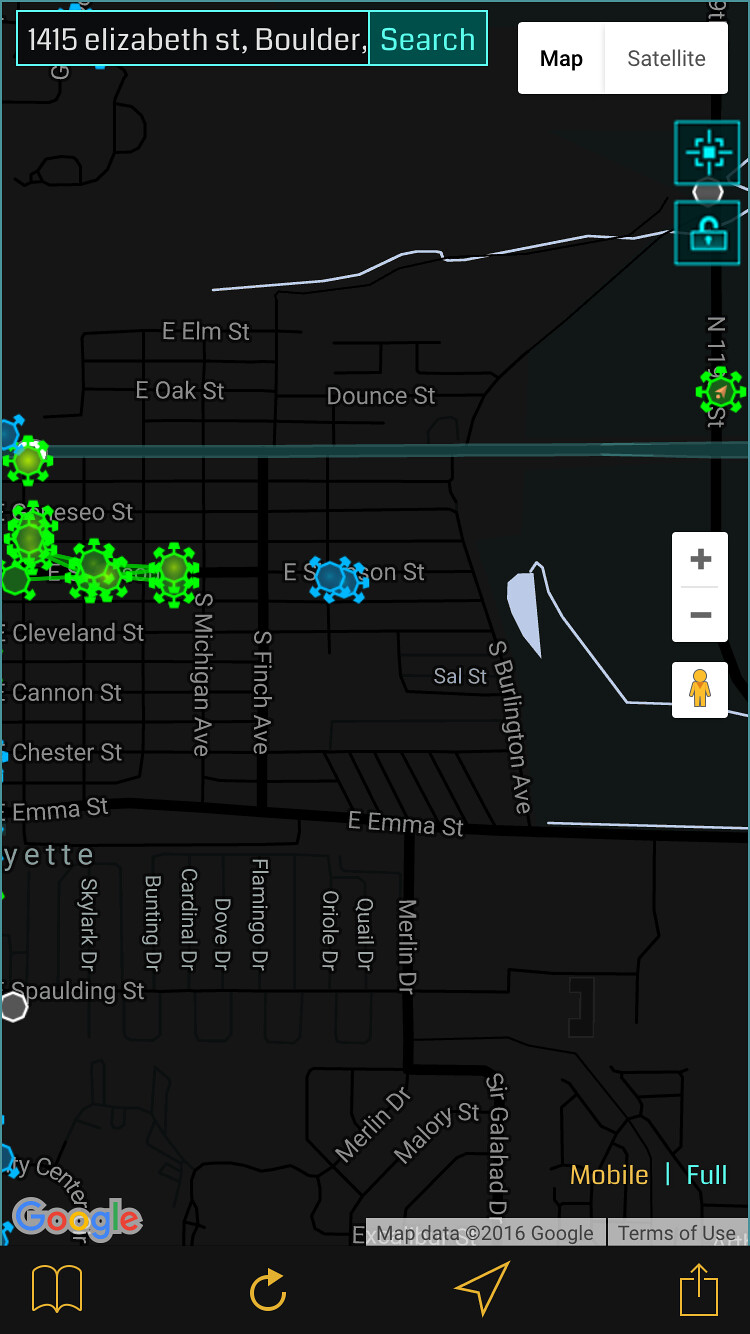This image is a detailed screenshot of a Google Map, specifically highlighting an address on Elizabeth Street in Boulder, Colorado. In the top-left corner, there is a turquoise and black search box displaying the queried address. The map mode used appears to be 'Satellite View' given the black background with streets delineated. Major thoroughfares, including a highway, are visible. Various markers with prongs extend off them, some in blue and others in green, possibly denoting different points of interest or locations. At the bottom-right corner is a small gray box that states "Map data ©2016 Google" along with a "Terms of Use" link. The precise location of the searched address is indicated by a distinct dot on the map, pinpointing the location within the larger geographic context.